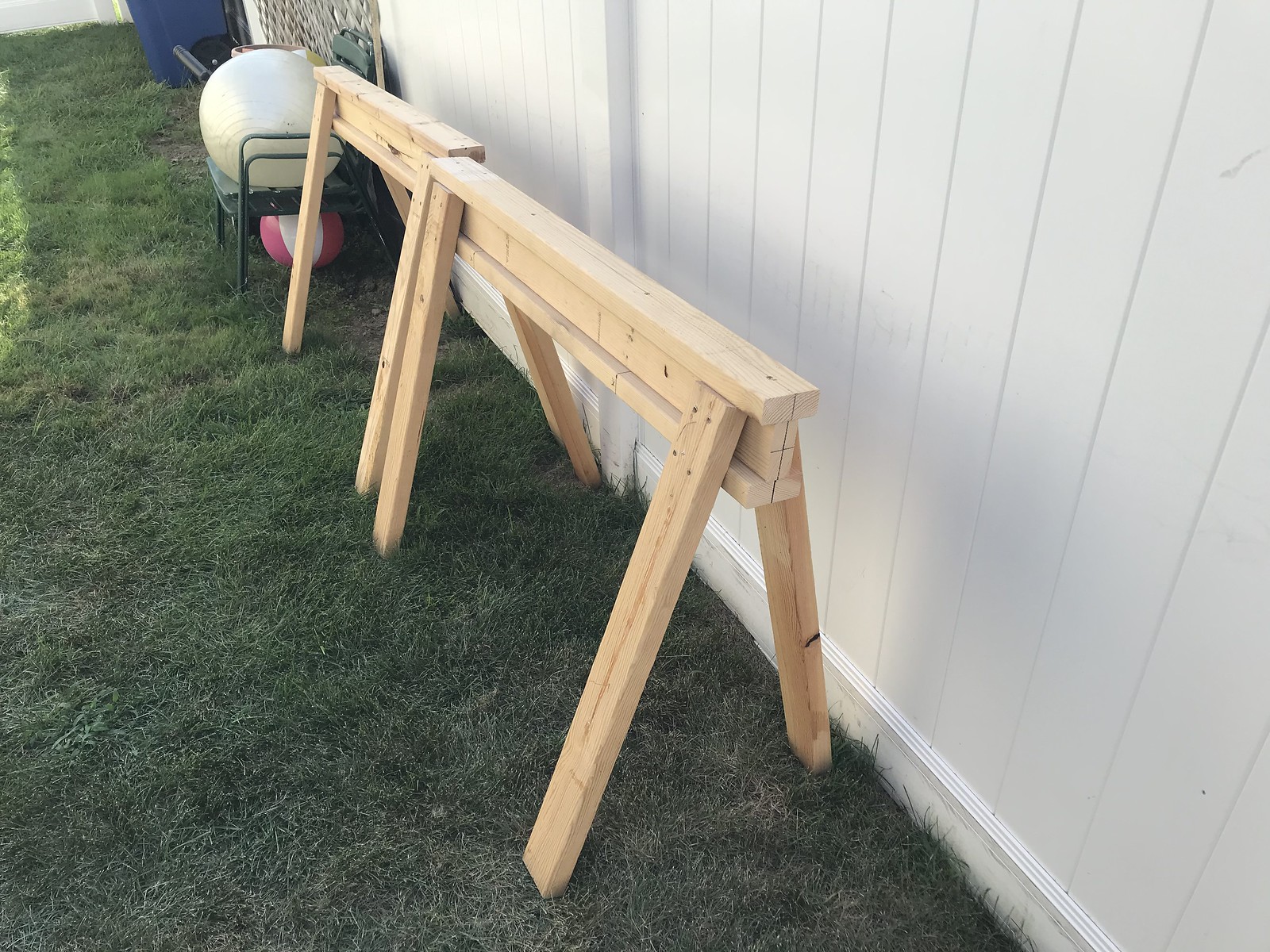This photograph, taken outdoors, captures a scene dominated by a large white privacy fence with vertical slats. In front of the fence, there are two freshly made wooden sawhorses constructed from unstained, unweathered 2x4s, with visible nails holding them together. These sawhorses are positioned side by side on a grassy lawn. Nearby, two green metal chairs are stacked, with a large white exercise ball resting on top. Underneath the chair, there's a pink and white ball, possibly a beach ball or volleyball. In the corner of the image, a blue plastic garbage bin with wheels is partially visible. There also appears to be some sports equipment scattered around, including netting that might be for soccer, and a navy blue object with a long pole. The right side of the fence transitions into a section of mesh or chain-link, providing a view of the yard beyond.